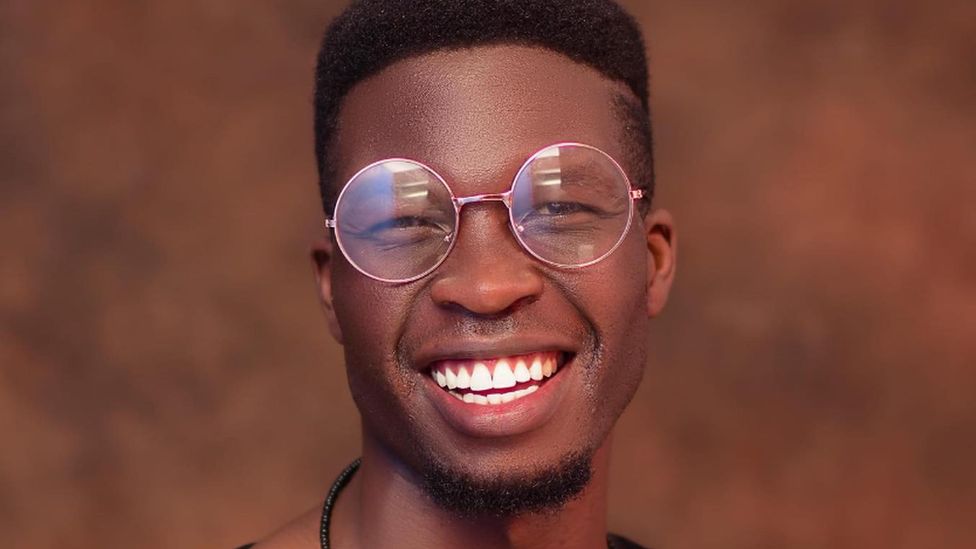The photograph showcases a young, cheerful black man with a big, friendly grin. His smile reveals perfectly white teeth, and he wears distinctive, round eyeglasses with unique silver or rose-gold frames that reflect some light. He sports a high-top hairstyle with the sides deliberately shaved, creating a dense cylindrical shape on top of his head. His facial hair is limited to a small goatee. Around his neck, a black leather thong necklace, possibly holding a pendant or medallion, is visible. The background is a mottled brown, slightly out of focus, complementing his skin tone. Thin eyebrows frame his expressive eyes, reinforcing his amiable and approachable demeanor. He is dressed in black, with only the portion of his neck and some parts of his shoulders visible in the frame.